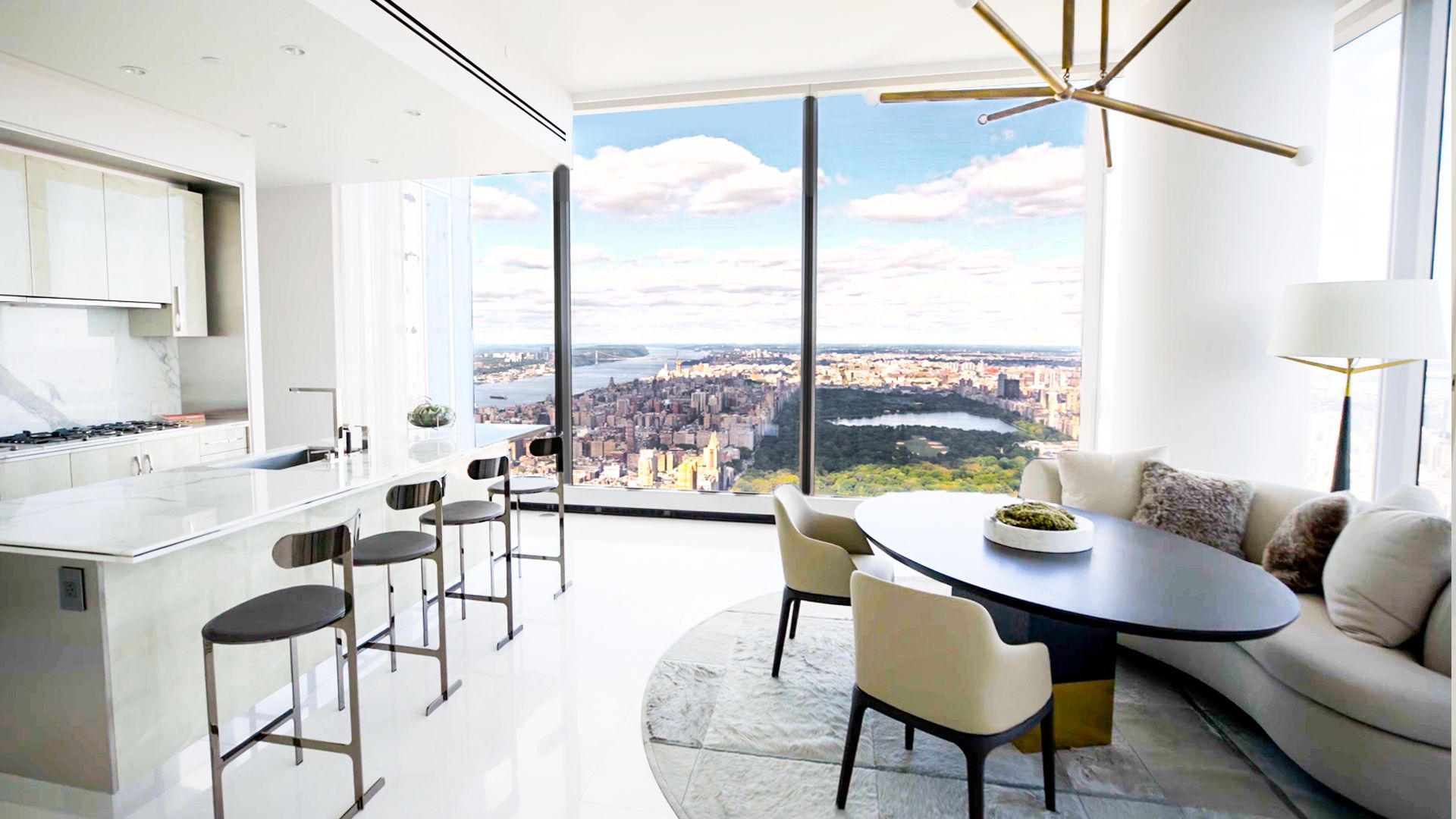This photograph showcases the interior of an upscale high-rise apartment, featuring a modern and elegant design predominantly in white. In the foreground, on the left side, there's a sleek bar area with a white marble countertop and four black bar stools featuring three-point bases. The bar setup includes a sink and is complemented by wall-mounted cabinets. To the right, the dining and seating area includes a long sofa with decorative throw pillows, flanked by an oval coffee table and two white chairs with black legs arranged across from it. Behind the sofa, there's a contemporary lamp, and the floor is adorned with a white rug featuring tile-like textures. Above, a modern art fixture serves as a light source. The far wall is dominated by floor-to-ceiling windows that offer a stunning view of Central Park, with a clear sight of the reservoir in shade, surrounded by sunlight, blue sky, and white fluffy clouds, looking towards the uptown area. The overall space is airy, filled with natural light, and accented by a few plants.